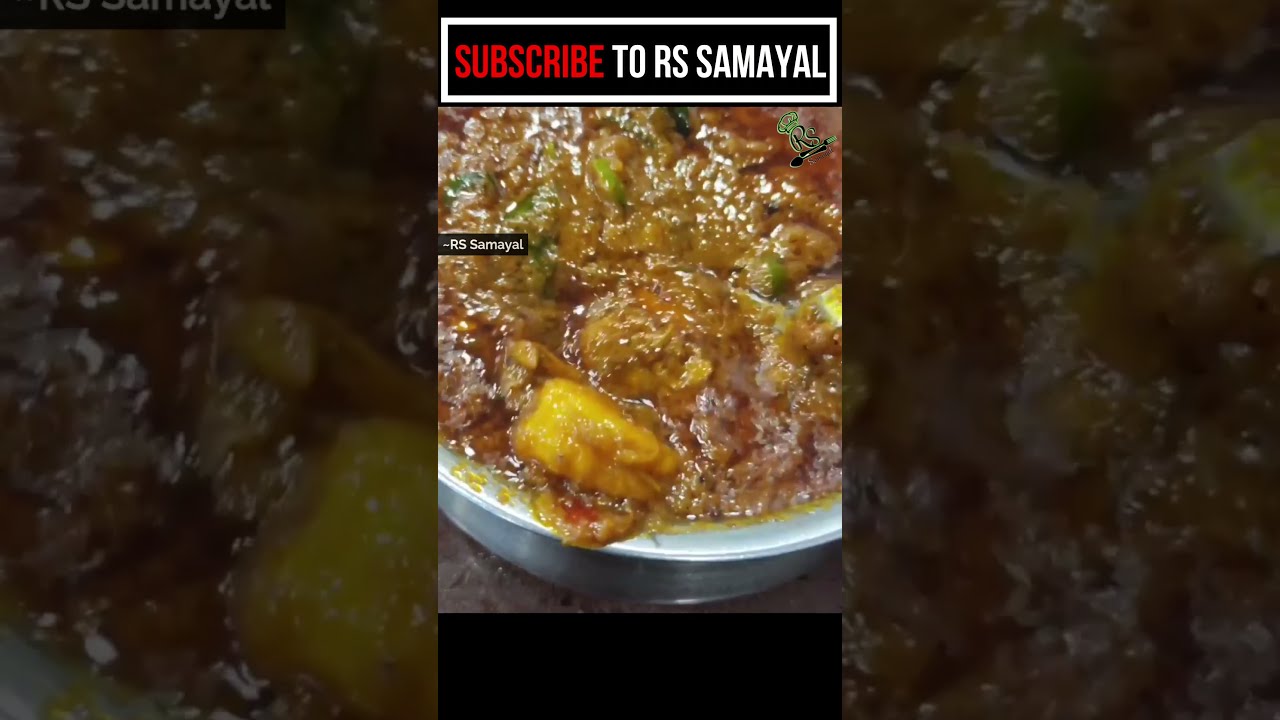This image, a screen capture likely from a TikTok video, features a detailed, up-close view of a hearty, simmering stew or curry in a silver dish. The top section of the image contains a prominent banner with a black text box outlined in white, instructing viewers to "subscribe to RS Samael" in red and white text. Accompanying this subscription message is a small logo with the initials "RS," adorned with a chef's hat, a spoon, and a fork. The main focus of the image is the stew itself, which is a rich brown color interspersed with vibrant ingredients. There are visible sliced green chili peppers and chunks of yellowish-orange chicken or shrimp, suggesting a spiced, flavorful dish. The surface is bubbling, indicating it is currently being cooked to perfection. The entire presentation is framed within a cell phone-sized focal area, surrounded by darker panels on the sides, highlighting the stew’s rich and vivid appearance.